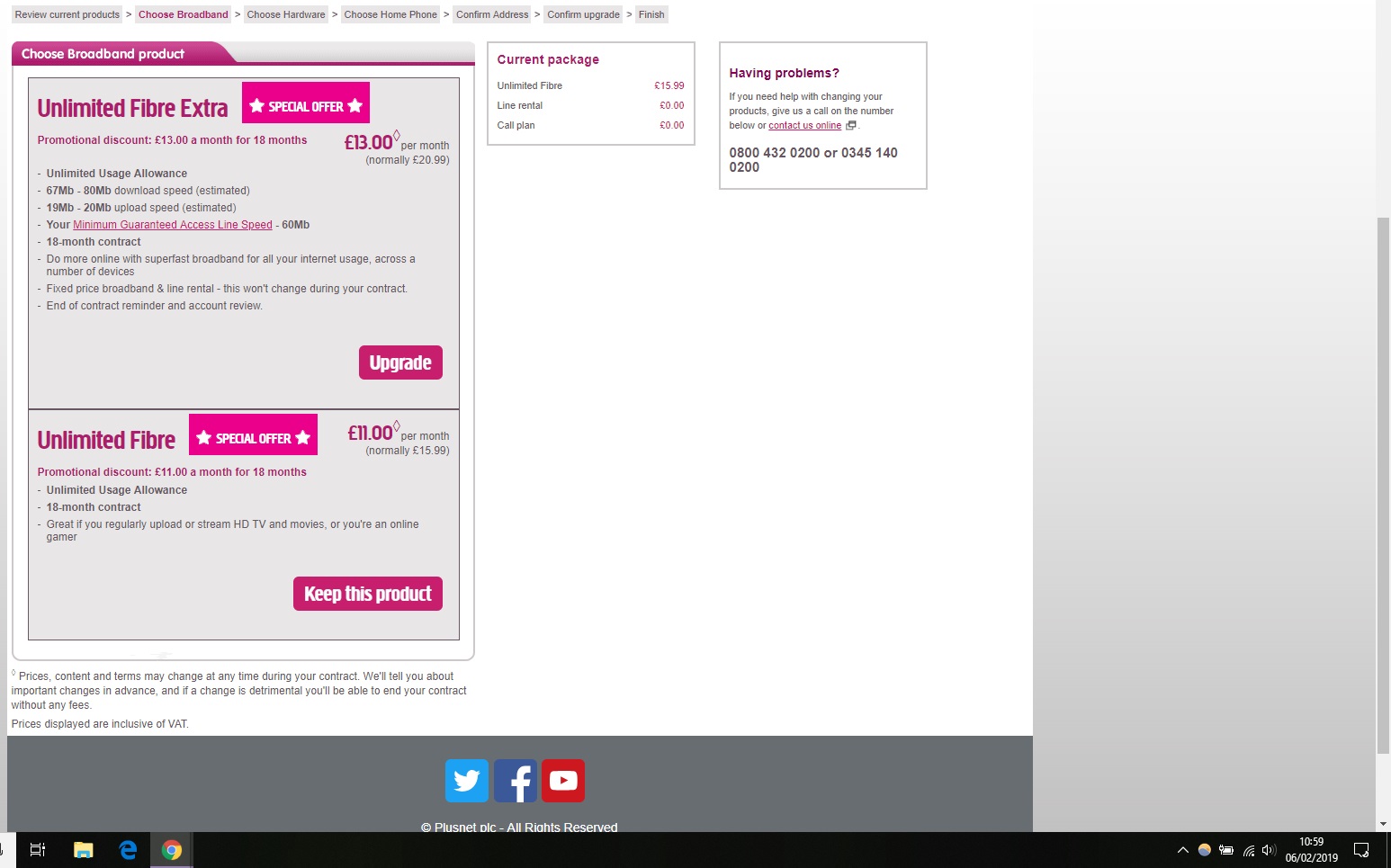Screenshot of Web Page for Choosing Broadband Plans

This screenshot captures a web page with a predominantly white background, accented with pink and black text. Key navigation steps are outlined at the top, listed as: "Review Current Products," "Choose Broadband," "Choose Hardware," "Choose Home Phone," "Confirm Address," "Confirm Upgrade," and "Finish." The "Choose Broadband" step is highlighted in pink, indicating the current stage in the process.

Beneath this, the section titled "Choose Broadband Product" presents two distinct options: "Unlimited Fiber Extra" and "Unlimited Fiber," both marked with a "Special Offer" banner. The "Unlimited Fiber Extra" option has an "Upgrade" button, while "Unlimited Fiber" has a "Keep This Product" button. Each option includes detailed descriptions of the features provided.

To the right, two informational boxes are displayed. The first box, labeled "Current Package," lists: Unlimited Fiber at $15.99, with Line Rental and Call Plan both at $0. The second box, titled "Having Problems?" offers assistance information, advising users to either call 0800-432-0200 or 0345-140-0200, or to contact support online if they encounter issues while changing products.